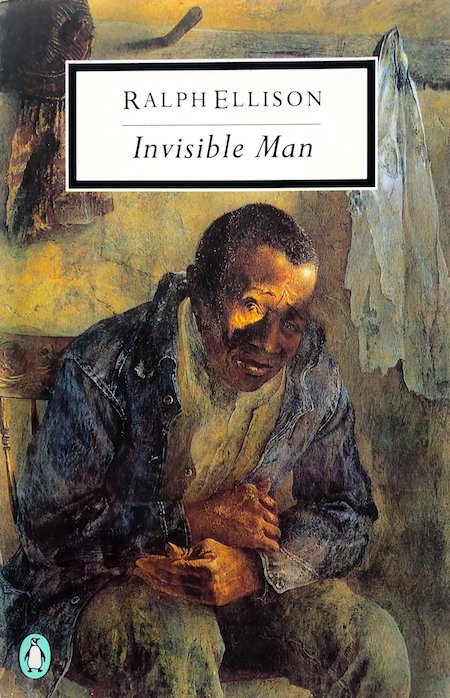The book cover of Ralph Ellison's "Invisible Man" features a detailed illustration of an African American man seated on a wooden chair. He is dressed in a blue denim jacket, white shirt, and dark pants, with his hands folded on his lap. The man's face is partly illuminated by light, highlighting his right eye, while his left eye remains in shadow, lending a contemplative and somber expression to his gaze. He appears to be looking directly at the viewer, his lips closed and eyes reflecting a sense of sadness. The backdrop includes a yellow wall adorned with a coat rack. Hanging on the rack are a white shirt and what appears to be a scarf. Above the man's head, the text "Ralph Ellison, Invisible Man" is prominently displayed in white lettering. The cover also features an image of a small penguin located in the bottom left corner, indicative of the publisher.